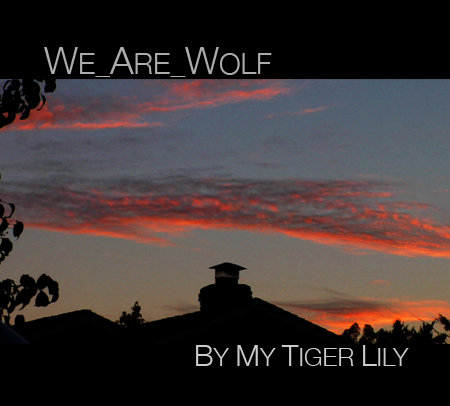The image resembles a CD cover with a square composition. The top portion of the cover features a black background with the text "we_are_wolf" written in white letters. The primary focus of the image is a beautifully dramatic sunset sky, dominating the upper two-thirds with a blend of vivid red and orange clouds against a grayish-blue backdrop. As the sky fades into darkness toward the horizon, silhouettes of buildings and trees emerge. These black silhouettes, which include details like the outlines of a house with a chimney and tree leaves, are artfully contrasted against the striking sunset. The bottom portion of the image continues this silhouette theme with more indistinct shapes of houses and trees. At the bottom right, the text "by_my_tiger_lily" is displayed in white letters, punctuating the dark silhouettes in the foreground.